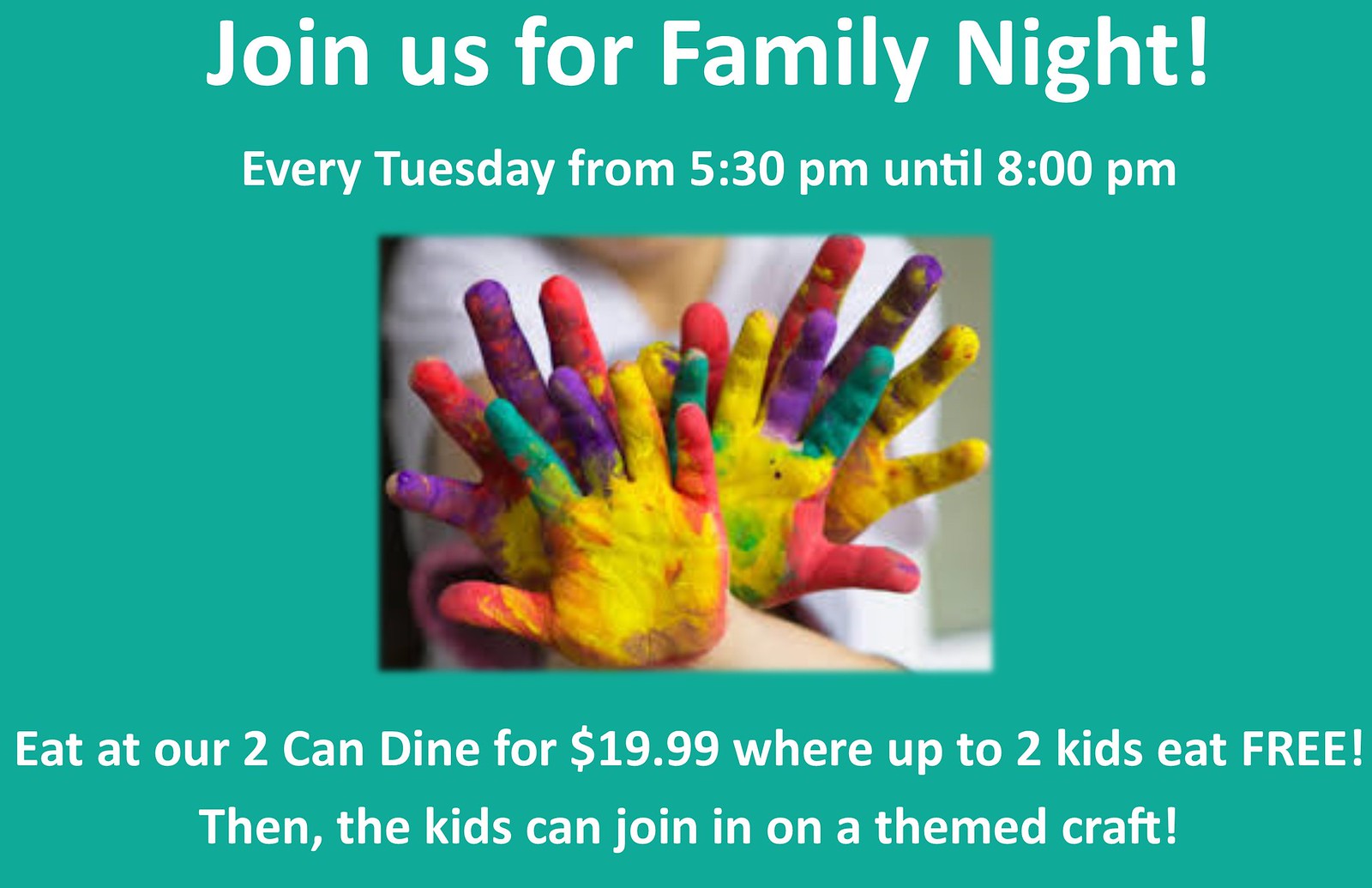The advertisement features a green background and a landscape orientation. At the top in white text, it announces "Join us for Family Night!" Below that, it states, "Every Tuesday from 5:30 p.m. until 8 p.m." The centerpiece of the ad is a rectangular image displaying four live child's hands, fully covered in vibrant paint colors including yellow, orange, green, purple, red, blue, and pink, held up towards the camera. Beneath the image, white text offers a dining deal: "Eat at our two-can dine for $19.99, where up to two kids eat free." The ad concludes with the information, "Then kids can join in on a themed craft." This visually engaging advertisement effectively promotes a family night at a restaurant, combining dining with a creative craft activity for children.